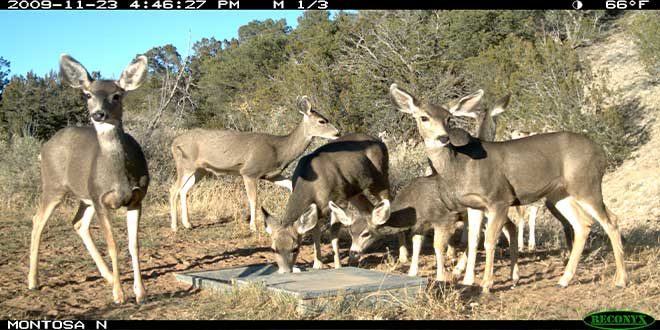The photograph, captured on November 23, 2009, at 4:46:27 p.m., in Montosa (likely in North Dakota), shows a group of five deer foraging together on a field with scrub brush and dried grass. The temperature was 66 degrees Fahrenheit at the time. The background includes trees, while the foreground features a man-made feeding area that the deer are gathered around, suggesting the animals might be on a preserve designed to support them. Two of the deer are looking directly at the Reconyx trail camera responsible for the image, evident from the logo on the bottom right corner. The still footage conveys a calm, overcast yet bright afternoon, immortalizing the natural behavior of these wild, antler-less deer.